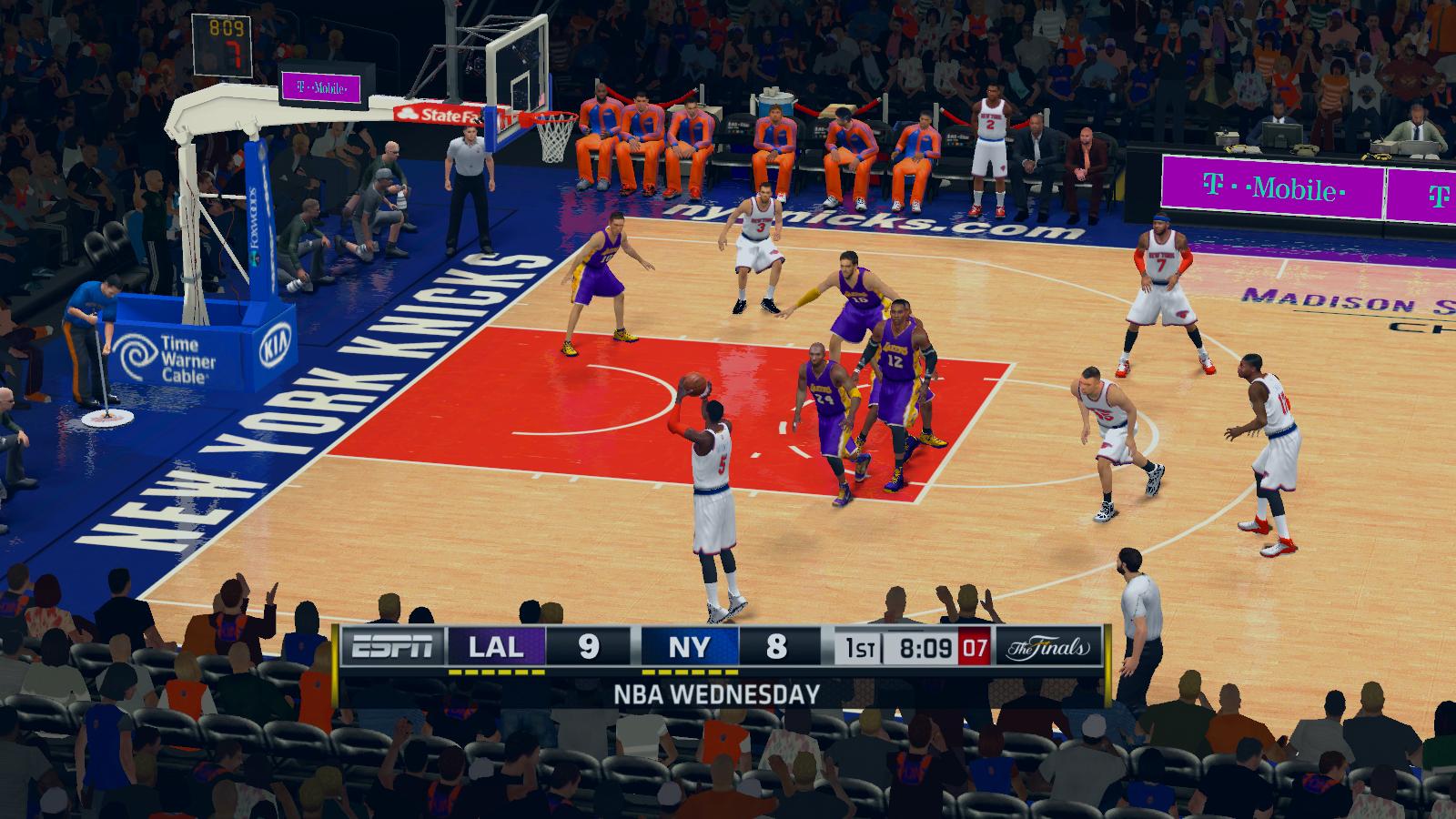The image is a detailed, simulated screenshot of an NBA basketball game broadcasted on ESPN, showcasing a match between the Los Angeles Lakers and the New York Knicks. The scoreboard at the bottom of the screen indicates that it's the first quarter with 8 minutes and 9 seconds remaining, and the score is 9-8 in favor of the Lakers. This is part of the NBA Wednesday finals. The game takes place in New York, depicted by the text "New York Knicks" on the court.

In the scene, players are in motion with one Knicks player preparing to take a shot. You can see five Lakers players, wearing purple uniforms, closely grouped together, while the Knicks players appear more spread out. Two referees are visible, positioned on the right and left top corners of the court. The Knicks' bench and players on the sidelines are observable in the background. Additionally, advertisements for State Farm and T-Mobile can be seen on the arm of the backboard and the sidelines, respectively. The stands are packed with fans at both the top and bottom of the image, adding to the vibrant atmosphere of the game.